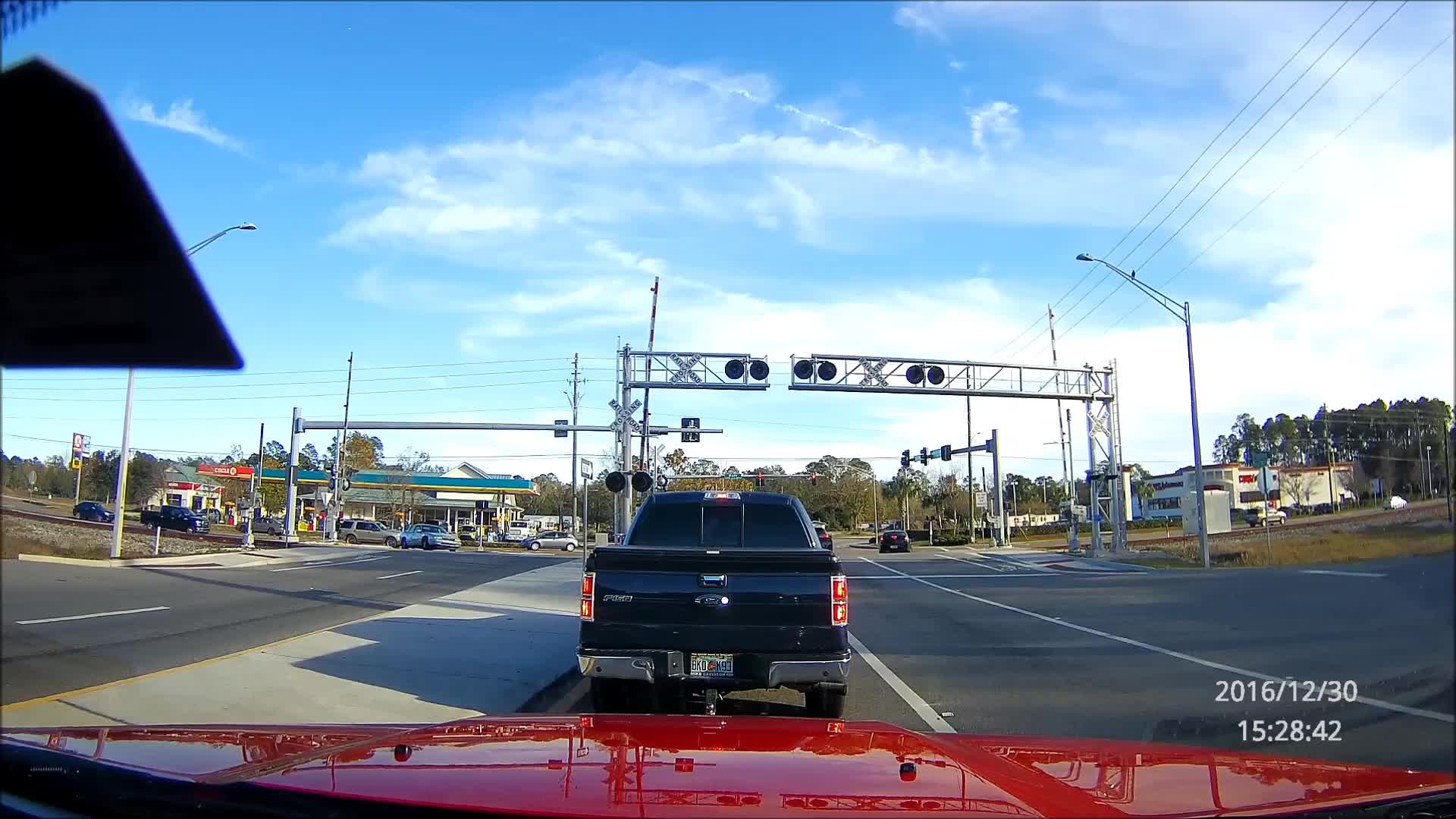The image is taken from inside a red car, likely by someone sitting behind the wheel, and looks out through the windshield onto a busy divided highway with at least two lanes on each side. Directly in front of the red car, there’s a black pickup truck, reminiscent of a Florida license plate on it. The photo captures a sunny day with some clouds in the sky. It's a busy road, approaching a significant intersection marked by large railroad crossing gates, indicating a railroad track ahead. The timestamp on the image reads "2016-12-30 15:28:42" in white ink at the bottom right corner. On the left side of the intersection are visible signs for a Shell gas station and possibly a BP station, confirming the bustling nature of the area. Power lines are seen on both sides, and the car’s driver's side sun visor slightly peeks into the frame.